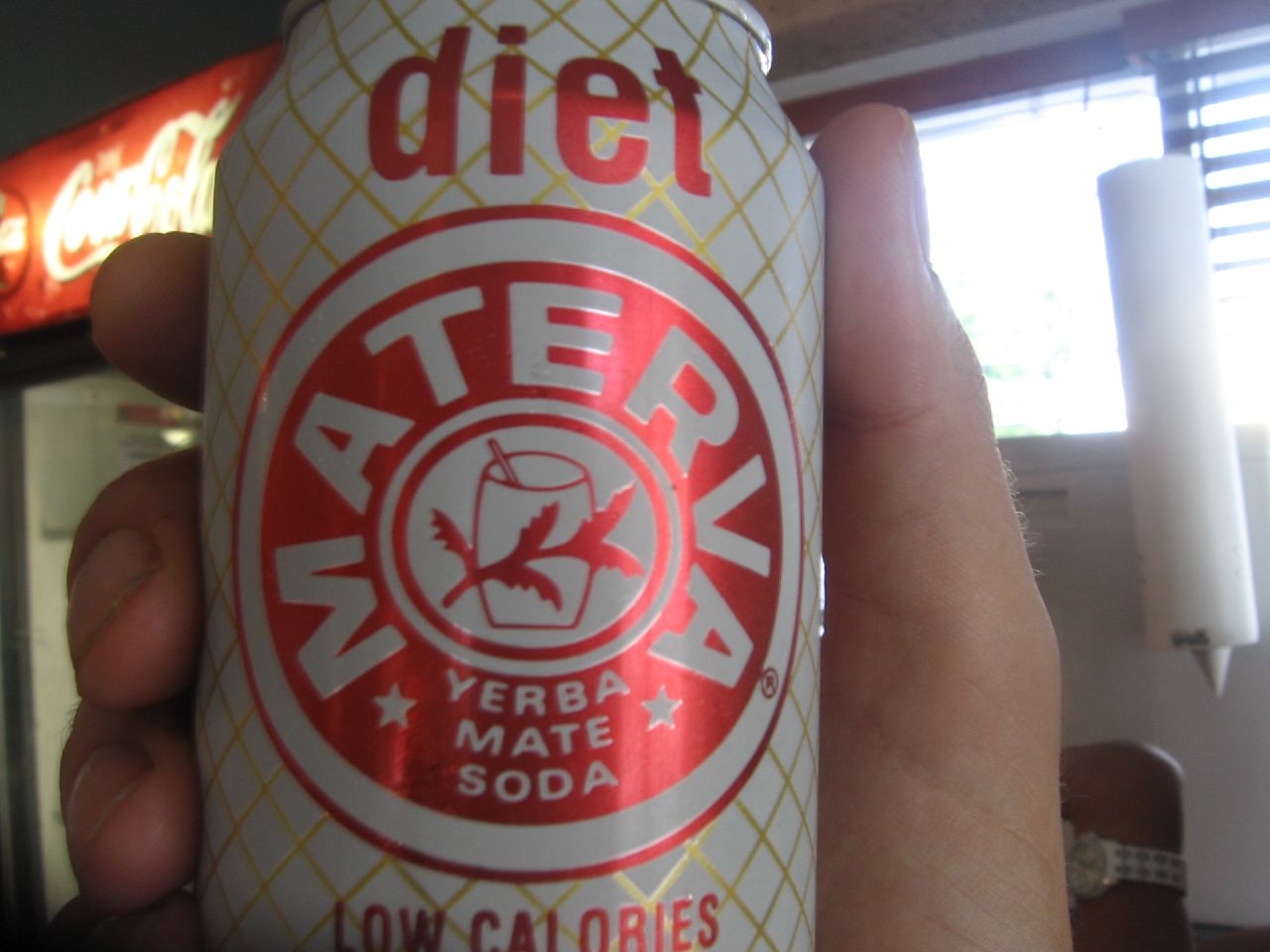A man's hand is prominently holding up an aluminum can of soda within what appears to be a convenience store or restaurant setting. The can is primarily white, adorned with a red and white logo, and features a crosshatch design with gold lines on the background. The text along the top of the can, in red, indicates that it is a diet soda. Upon closer inspection, the central part of the can displays a circular red logo with the white text "M-A-T-E-R-V-A" and two stars flanking the letters "M" and "A," all arcing within the circle. Inside the red circle, there's another white inset featuring a red illustration of a slightly rounded cup with a straw, accompanied by a depiction of a plant, signifying that it is a Yerba Mate soda. The bottom of the can has red text declaring "low calories."

In the surroundings, a transparent plastic container filled with pointed paper cups is noticeable. The left side of the frame shows a couple of window panes, letting some light into the space. Additionally, a Coca-Cola cooler is partially visible in the background on the left side, just behind the man's hand, adding context to the setting.